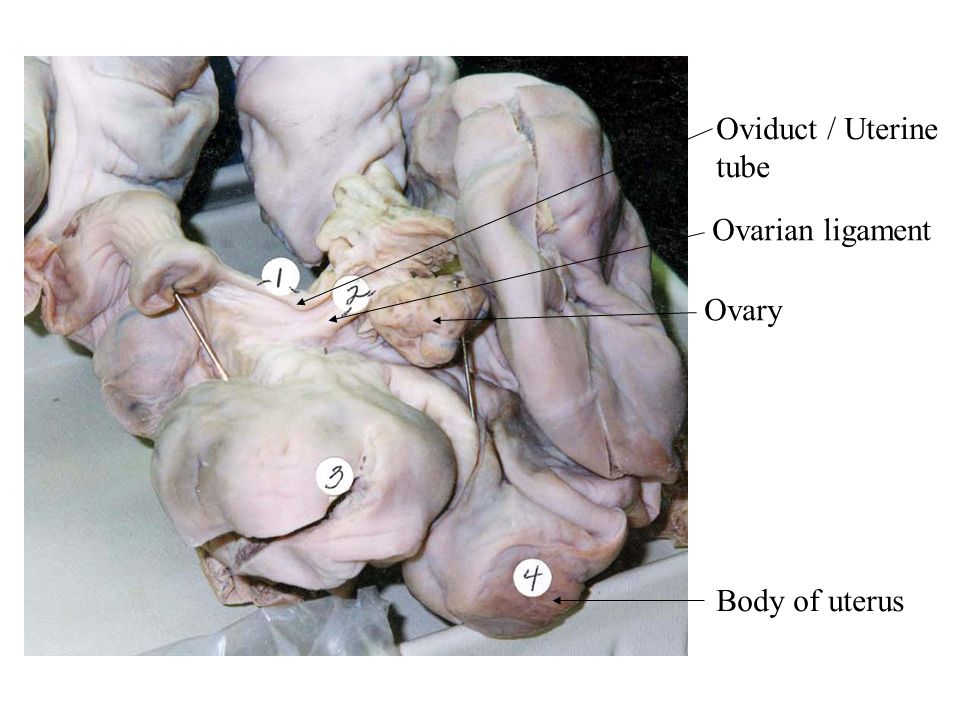This image displays anatomically detailed, labeled diagrams of female reproductive organs laid on a neutral-hued surface, likely white. The organs are a pale pink-brown and notably textured. Each organ is annotated with numbers 1 through 4, which are linked to the corresponding labels via black lines. Number 1 marks the "oviduct/uterine tube," positioned at the topmost part of the image. Number 2 identifies the "ovarian ligament" slightly below. Number 3 is labeled as the "ovary," situated lower still. Finally, Number 4 denotes the "body of the uterus," found at the very bottom of the arrangement. These anatomical parts are clearly displayed and highlighted for educational reference, emphasizing the reproductive systems with precise and structured labeling.